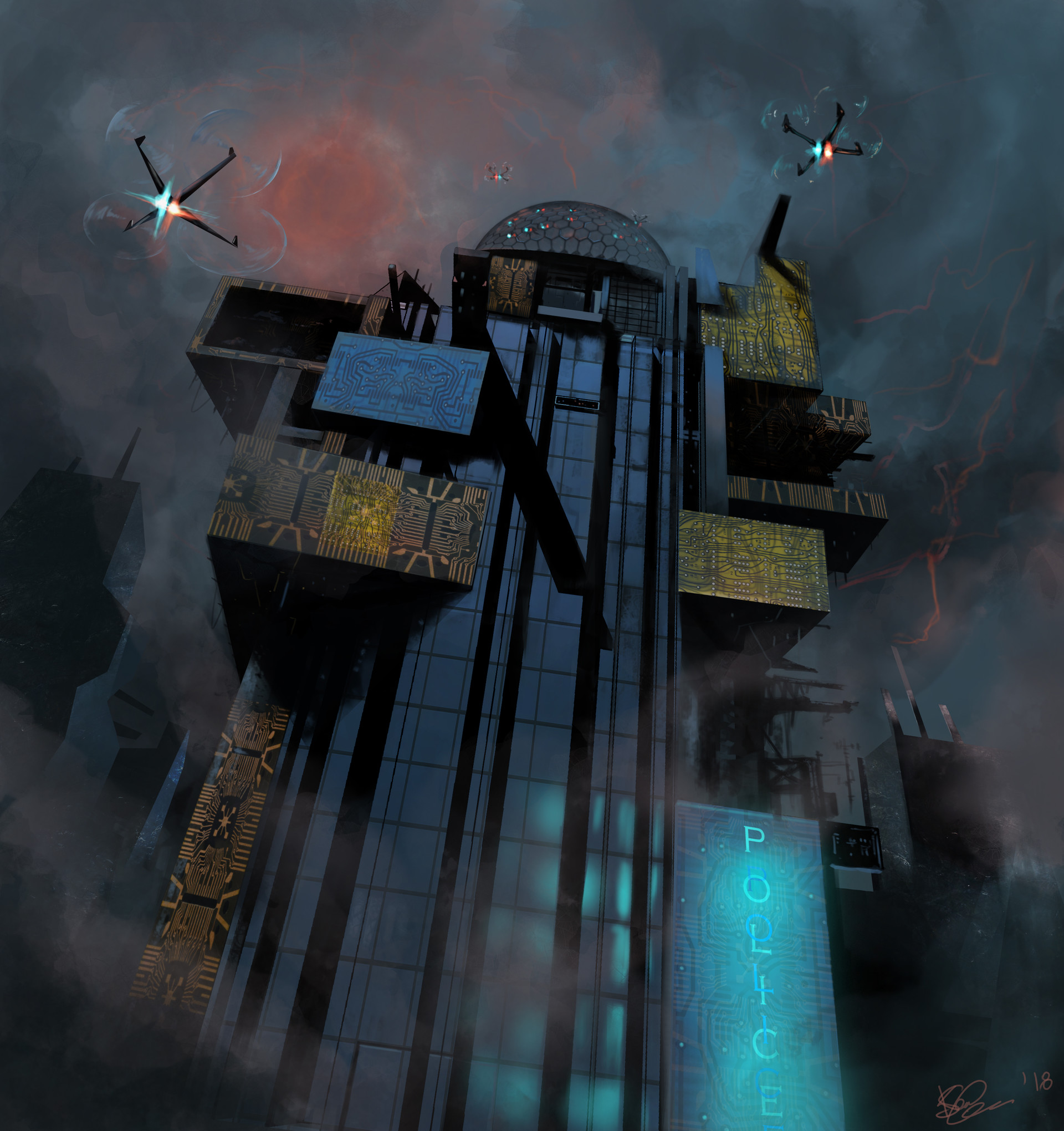The image is a highly detailed piece of digital artwork with a dark, futuristic theme. In the scene, two drones, each with wings shaped like an ‘X’ and equipped with swirling propellers, are positioned in the upper corners—one in the upper left and one in the upper right. Each drone features distinct red and blue lights. The focal point is a towering black building that ascends from the bottom center to the top of the image. This towering structure is adorned with intricate, ornate gold patterns that resemble circuitry designs, particularly visible on the top balconies. A prominent neon blue sign vertically spelling out “POLICE” is affixed near the building's base.

The environment around this structure is equally dramatic: an ominous sky filled with dark, turbulent clouds pervades the background. A sinister reddish glow permeates the upper left corner, suggesting a malevolent source of light, while red lightning streaks through the clouds in the upper right quadrant. The entire scene is engulfed in a dark and eerie atmosphere, magnifying the sense of a dystopian future.